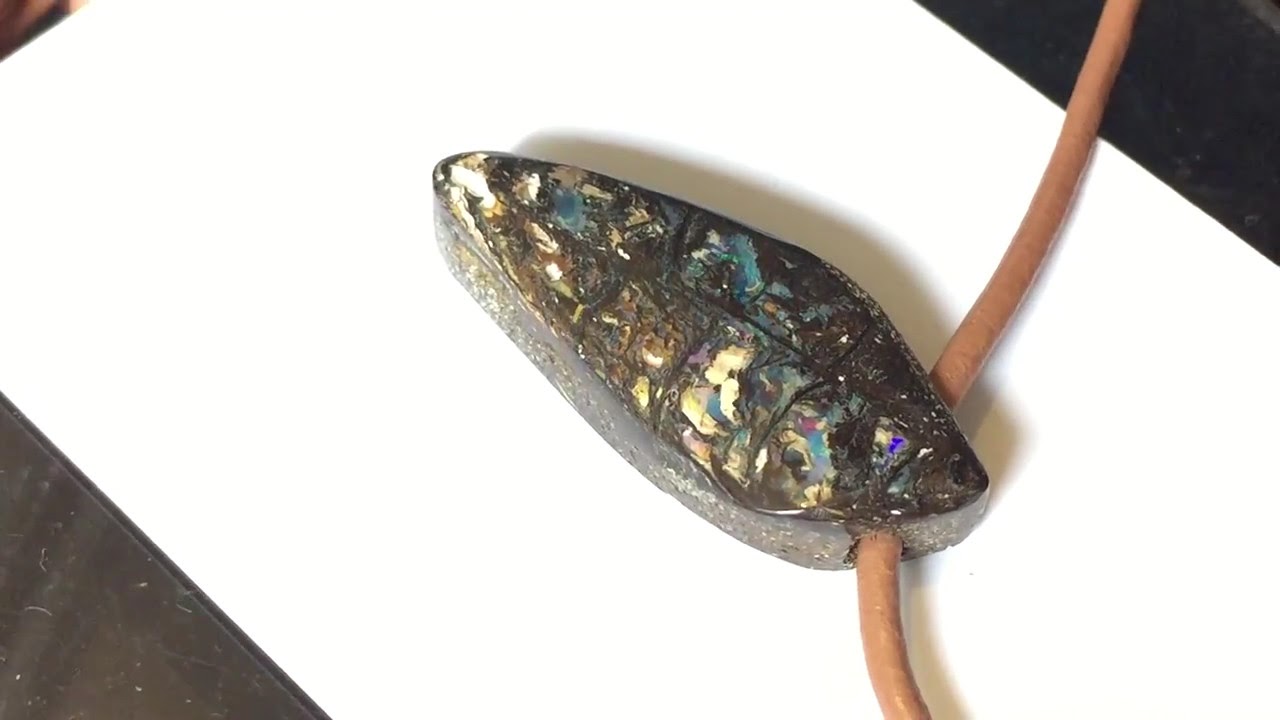The image depicts a necklace featuring a carved stone pendant attached to a thick brown leather band. The pendant, shaped like a leaf or possibly a tooth, is primarily green with a mix of other colors that give it a shiny, opalescent quality. The stone has a hole through which the band is strung. The entire piece is set against a white rectangular area, which in turn rests on a dark surface. The lighting in the scene originates from the lower left, casting a shadow of the pendant to the upper right.